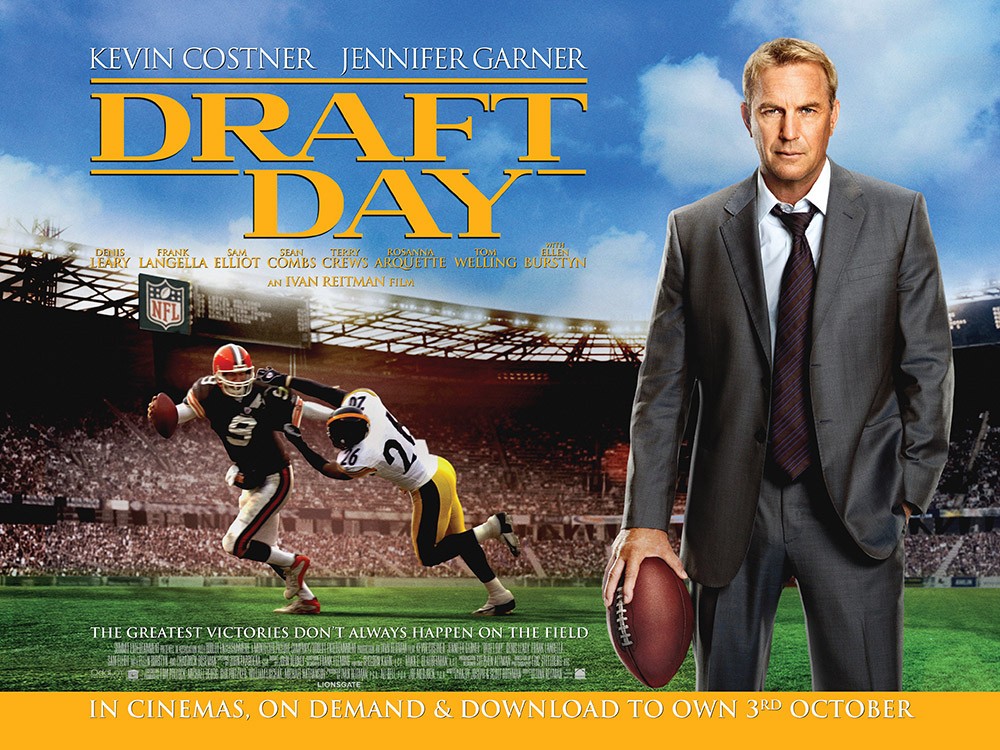This movie poster for "Draft Day" prominently features Kevin Costner on the right side, wearing a gray suit with a maroon tie and holding a football. He stands against a backdrop of a bustling stadium, packed with cheering fans and with bright stadium lights illuminating a semi-cloudy blue sky. The title, "Draft Day," is displayed in large bold yellow letters across the top left corner. Above the title in white letters are the names of the leading actors: Kevin Costner and Jennifer Garner.

Below the title, a football scene unfolds showing two players in action: a Cleveland Browns quarterback, recognizable by his orange helmet, brown jersey with a white number nine, and white pants with orange and brown stripes, is being tackled by a Pittsburgh Steelers defensive player, donned in a black and yellow helmet, white jersey with a black number 26, and yellow pants with a black stripe. The scene plays out on a vivid green field with a large full stadium in the background, also featuring a sign that says "NFL" near the stadium lights.

Accompanying the dynamic imagery are the words in white: "The greatest victories don't always happen on the field," prominently displayed near the green grass foreground. Below the main image, a gold horizontal bar contains white text that reads, "In Cinemas, On Demand, and Download to Own 3rd October." Additionally, credits for other stars like Dean Dennis Leary, Frank Langella, Sam Elliott, Sean Combs, Terry Crews, Rosanna Arquette, Tom Welling, with Ellen Burstyn, and an Ivan Reitman film, are also mentioned in small yellow letters below the title.